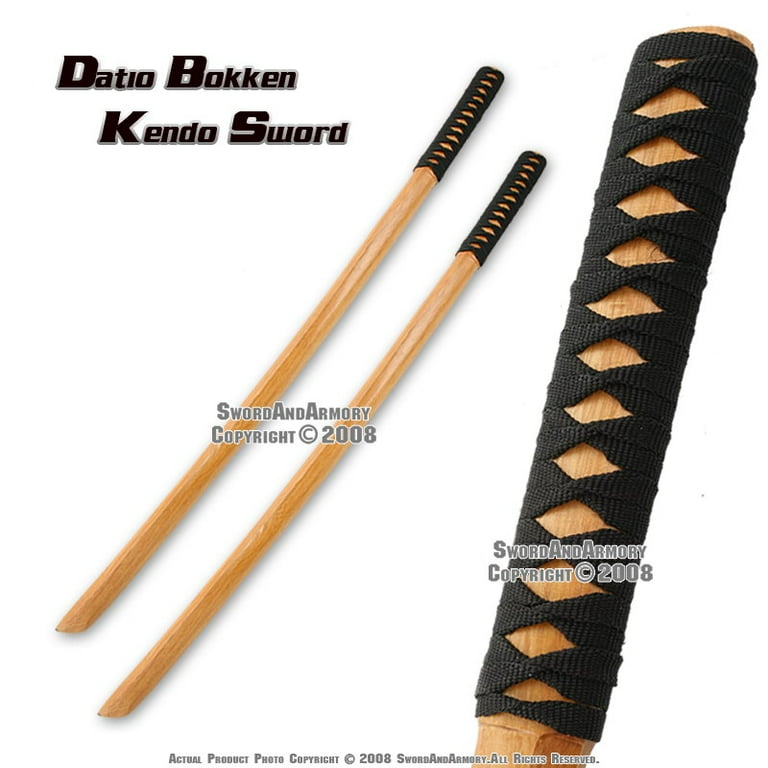This detailed advertisement showcases a Datio Bokken Kendo Sword against a completely white background. The image features two light natural wood-colored wooden swords placed diagonally across the center, both appearing blunt, without sharp blades. To the right, there's a close-up of the handle, which is intricately wrapped in a black fabric with a line of diamond-shaped holes exposing the wood beneath. Inscribed across various parts of the image, in black writing, is the text "Sword and Armory, Copyright 2008," and at the bottom, it states, "Actual Product Photo, Copyright 2008, Sword and Armory, All Rights Reserved."